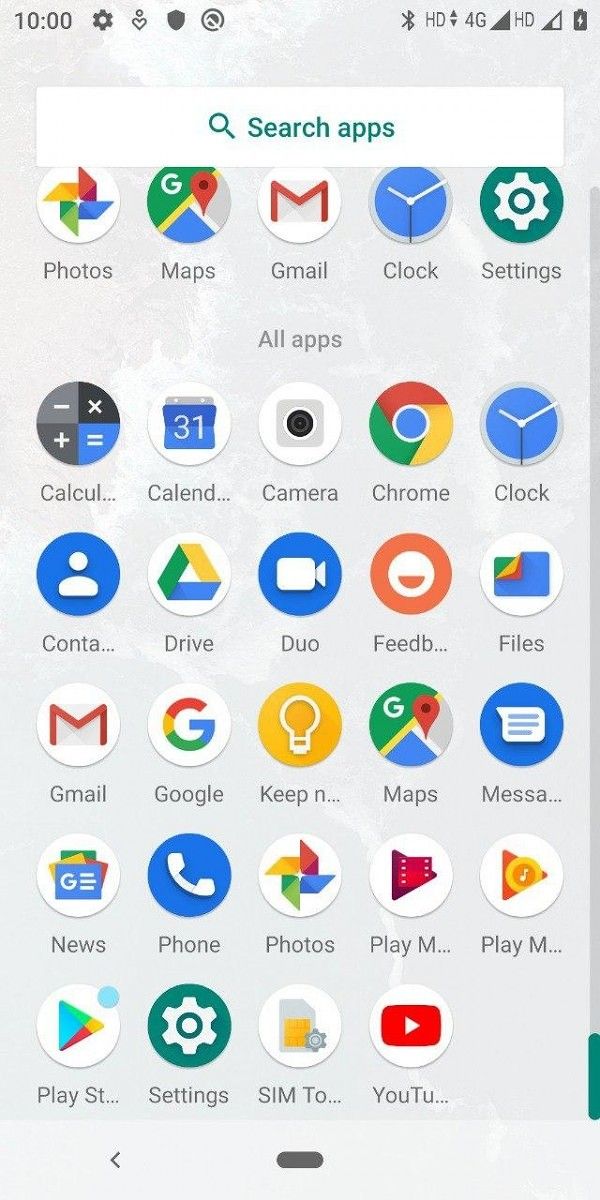The image depicts a smartphone's home screen, featuring multiple distinct elements and icons. The time is displayed at the top center, indicating 10:00. Various status icons are present along the top, including a gear icon (likely for settings), a heart icon, a shield icon, a checkmark within a circle, a Bluetooth icon, and network indicators like "HD," "4G," and "HD" again, this time showing about a 50% signal. The battery icon on the far right shows a nearly full charge.

Beneath the status bar is a search field with a magnifying glass icon, prompting users to "search apps." Directly below this field are five main app icons arranged horizontally: Photos, Maps, Gmail, Clock, and Settings, each with corresponding text labels.

Further down the screen, there is an organized grid layout displaying a variety of app icons, five across and five down, under the heading "All apps." Some of the visible apps include: Calculator, Calendar (with ellipsis indicating truncated text), Camera, Chrome, Clock, Contacts, Drive, Duo, Feedback, Files, Gmail, Google, potentially Keynotes, Maps, Messages, News, Phone, Photos, Play Music, Play Store, Settings, SIM Toolkit (abbreviated), and YouTube.

On the right side of the app grid, there is a large gray scroll bar, indicating the presence of more apps beyond the visible area, with a small green scroll marker at the very bottom. A back arrow is positioned at the bottom left corner of the screen, providing navigation options.